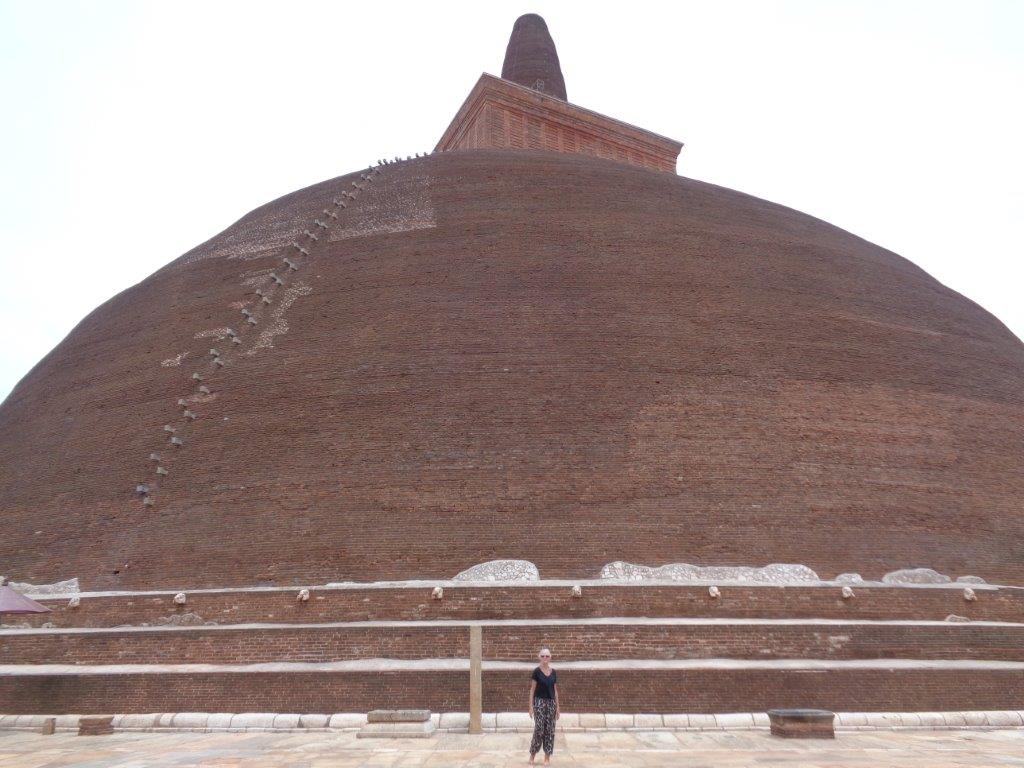The image depicts a striking outdoor scene featuring a massive, historical dome-like structure, predominantly composed of dark brown and red bricks, with white accents near its base. The structure, reminiscent of Roman architecture, dominates the center of the frame and is at least five to six times taller than the person situated at the bottom center. This person, an elderly woman wearing a black V-neck t-shirt, pants, white shoes, and sunglasses, stands on a stone walkway facing the camera, highlighting the immense scale of the dome behind her. Above the dome is a square, Roman-esque building structure topped with a smaller, rounded stone pillar. The sky is visible at the top of the image, adding to the open, expansive feel of the scene, indicative of a visit to a significant historical site. The colors in the image feature hues of blue, white, various shades of brown, and hints of off-red.